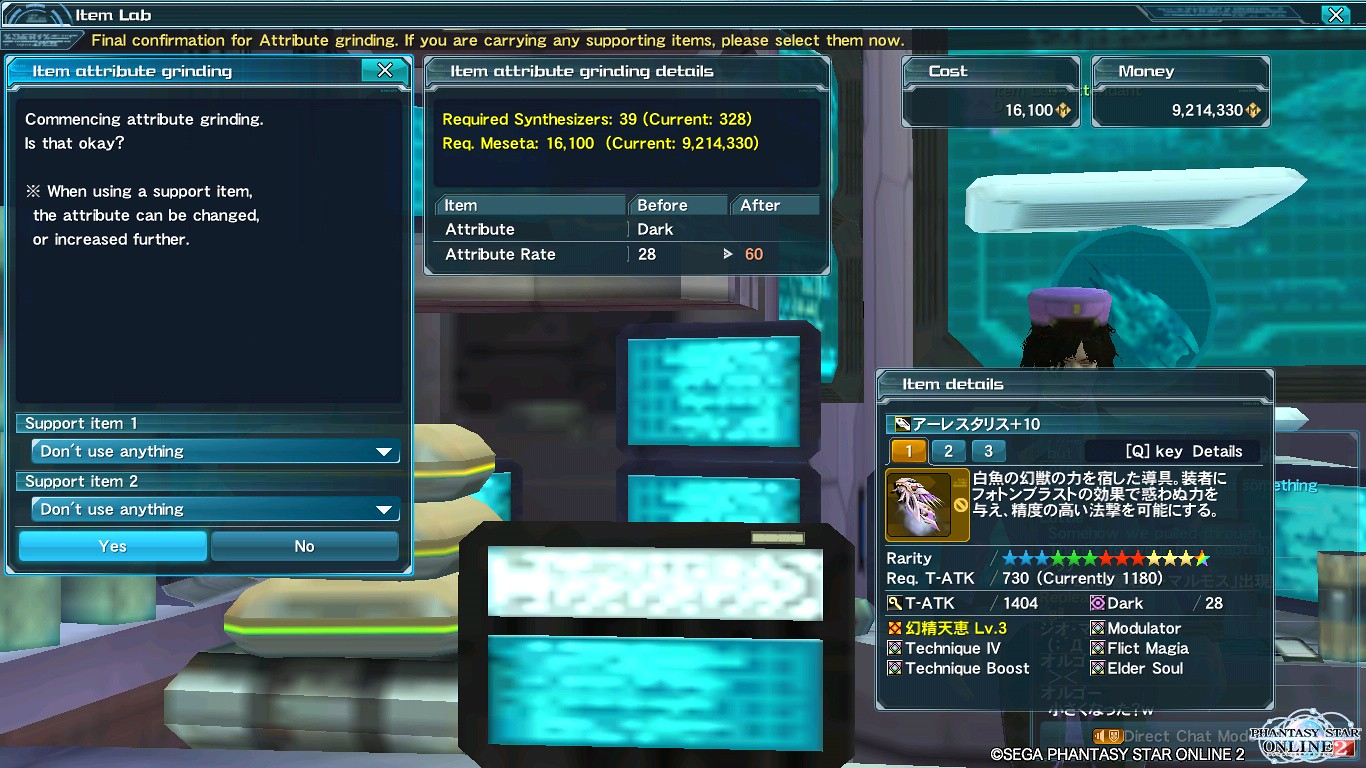The image is a screenshot from the video game "Phantasy Star Online 2," displaying a user interface for item attribute grinding. The screen prominently features a blue color scheme with futuristic, neon designs. In the upper left corner, a square box labeled "Item Attribute Grinding" contains a white prompt: "Commence Attribute Grinding, is that OK?" Below this box are options for selecting support items, "Support Item 1" and "Support Item 2," with dropdowns defaulting to "Don't use anything." The confirmation choices "Yes" (highlighted in light green) and "No" are at the bottom.

In the middle of the screen, a rectangular window titled "Item Attribute Grinding Details" provides specifics about required materials: "Required Synthesizer: 39, Current: 328" and "Required Meseta: 16,100, Current: 9,214,330." The right side of the screen includes smaller boxes labeled "Cost" and "Money." A partially visible character, seemingly a female figure with a blue headpiece, appears on the left side of the image. Additional text and a copyright logo can be seen in the bottom right corner, stating "SEGA Phantasy Star Online 2" in white, with the game's logo, where the number "2" is highlighted in red and white. Text in an Asian language, possibly Japanese, further details item attributes in various sections of the screen.